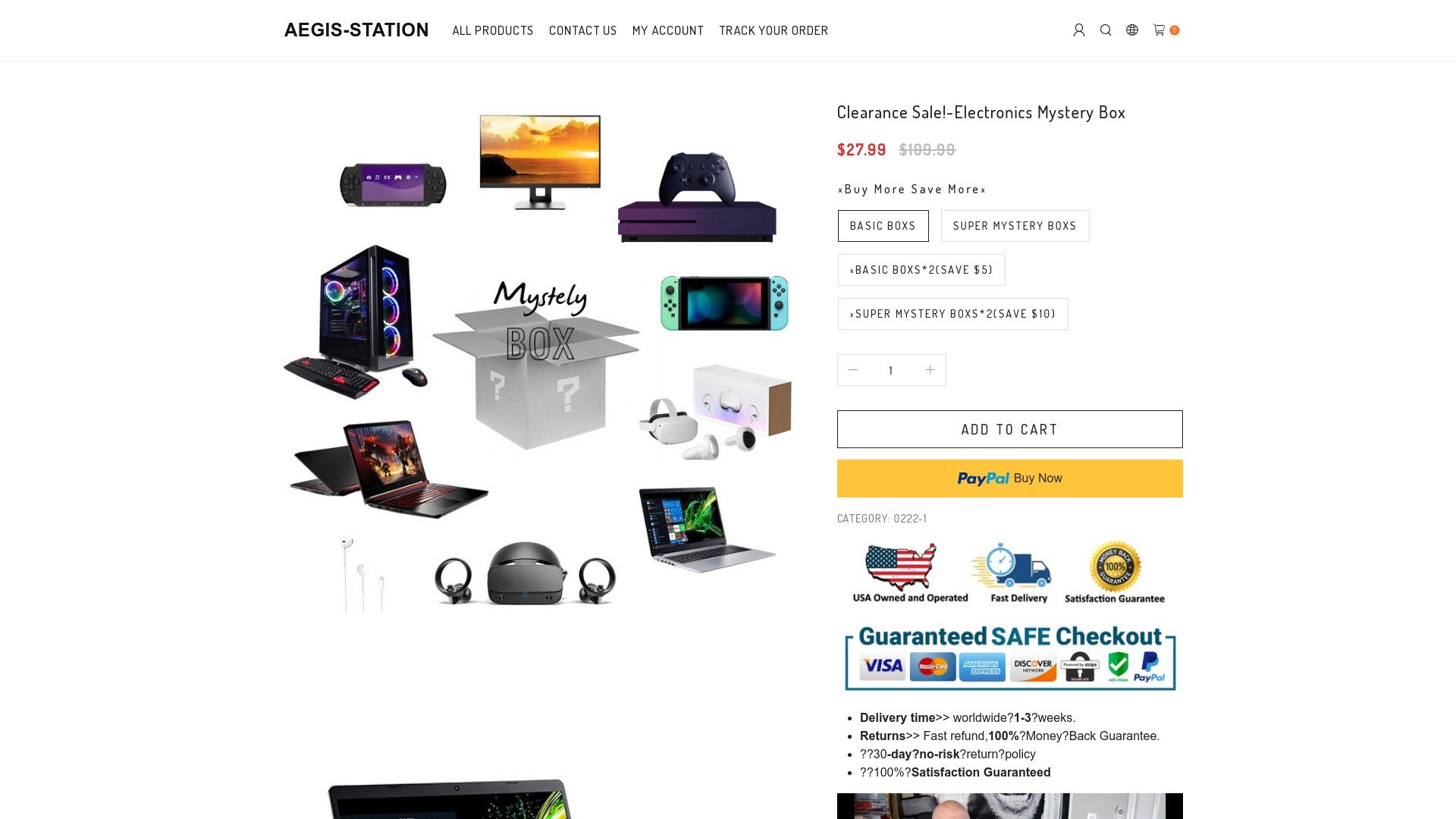This is a screenshot of an electronics retail website named AEGIS-Station. The interface features a navigation menu at the upper right corner, offering quick access to 'All Products,' 'Contact Us,' 'My Account,' 'Track Your Order,' 'Profile,' 'Search,' and 'Cart' options, depicted by icons.

On the left side of the homepage, product images are arranged in a circular layout around a central grayscale box labeled "Mr. Lee box," which appears to be a typographical error for "Mystery Box." The mystery box is adorned with question marks, suggesting surprise contents.

Products displayed include:
- A monitor (top position)
- A gaming console
- A handheld gaming device
- Three VR headsets with controllers
- A laptop
- Additional VR headsets
- Two more laptops
- A gaming PC
- Another handheld device

To the right of this display is a promotional section highlighting a "Clearance Sale Electronics Mystery Box" with an original price of $2,799, now marked down from $100, indicating a significant discount. There are different options for purchase, including basic and super mystery boxes. The basic boxes offer a $50 savings, while the super mystery boxes provide a discount of approximately $100 or $101. Options for purchasing include 'Add to Cart' and 'PayPal Buy Now.'

Further details include:
- A U.S. map graphic indicating that the service is "U.S. owned and operated" with promises of "fast delivery" and "satisfaction guaranteed."
- Icons for various credit cards suggesting secure checkout options.
- Additional tags concerning delivery times and return policies.

There are also a couple of JPEG images below the main content area, though they are partially cut off and their details are indiscernible.